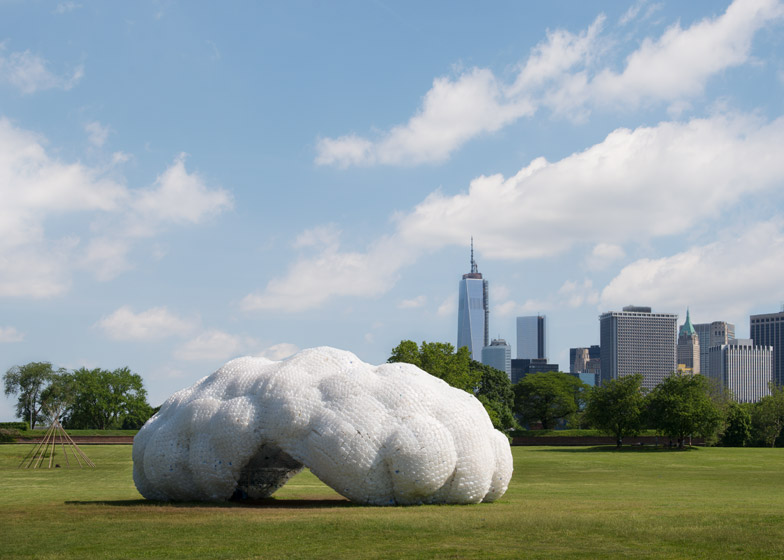The image captures a vibrant outdoor scene on a bright, sunny day with a sky of clear blue and sporadic fluffy clouds. The foreground is dominated by a peculiar white sculptural structure, lumpy and textured like a cloud, situated in a grassy plain. This large, intriguing sculpture features an archway in the middle, inviting the possibility of wandering through it. Adjacent to the sculpture is a teepee-like or pyramid-shaped structure made of sticks. Behind these central elements, a line of darker green trees frames the view, while further in the background, a city skyline with tall, distinct skyscrapers, including one with a pointed top, is visible. The entire scene is well-lit, with the crisp clarity of the day enhancing the contrast between the natural and man-made features.